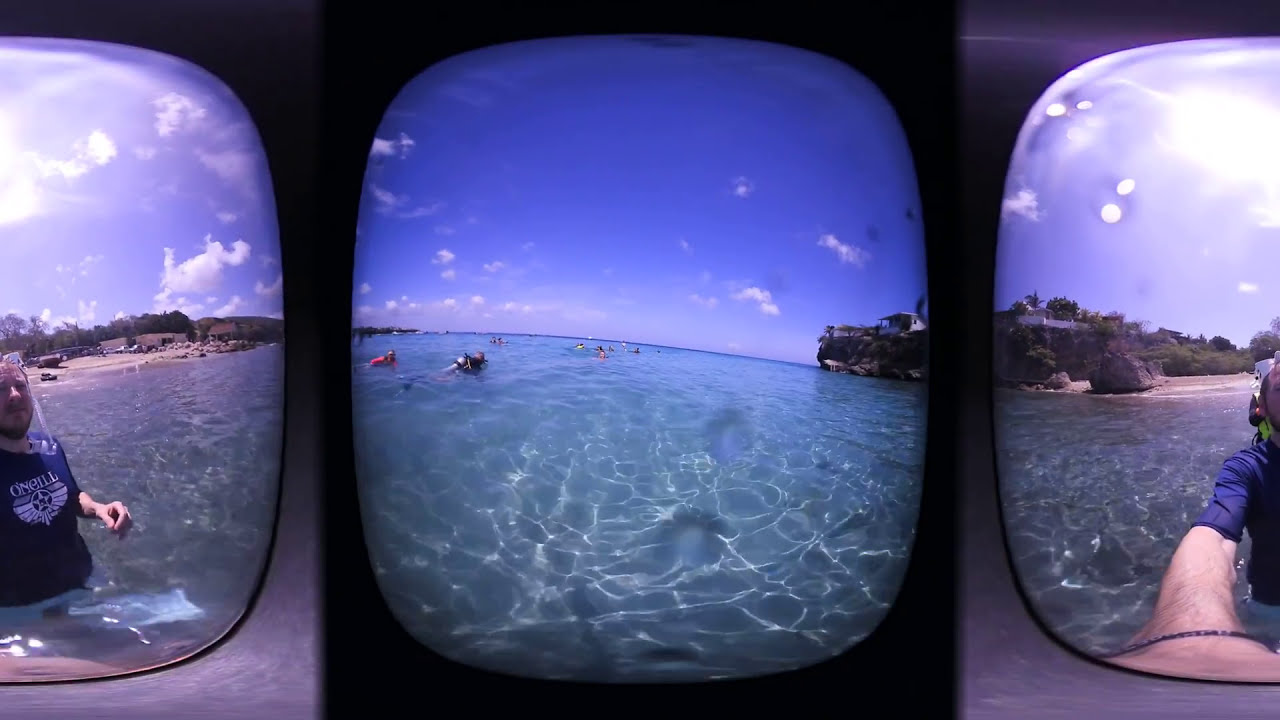The image is a triptych view, resembling a scene seen through airplane windows, comprised of three distinct sections, each displaying a part of a broader outdoor landscape. On the left, there is the right half of a person's face and upper torso, an older individual with grayish hair, wearing a white shirt adorned with a design featuring wings and a wheel. This person's right arm is outstretched, holding a camera lens. The middle section reveals a clear, waist-deep body of water, possibly an ocean bay or a pool, with several snorkel scuba divers and people in safety vests swimming. The sky above is a dark purplish-blue with some clouds near the horizon. On the right, the person’s outstretched arm meets a sliver of overexposed sky, and a dark cliff with a white building atop emerges, framed by a lush, green hill and part of a sandy shoreline. The colors in the image range from black, gray, blue, white, tan, light blue, to green, capturing a vibrant midday setting in an outdoor, aquatic environment.